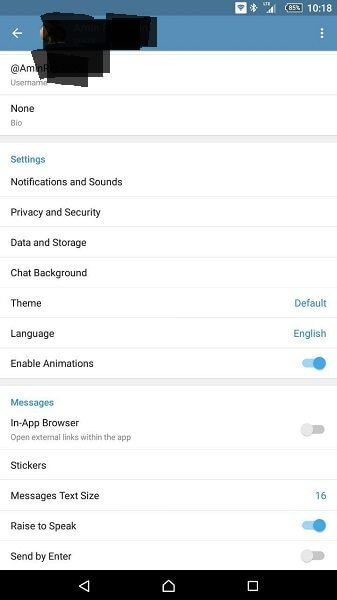This is a screenshot of a mobile application's settings interface. 

At the very top of the screen, the username is displayed prominently. Directly below that, the text "none8p" is visible. The user has navigated to the "Settings" section, where several options are organized in a list. The options displayed are as follows:
 
1. **Notifications and Sounds**
2. **Privacy and Security**
3. **Data and Storage**
4. **Chat Background**
5. **Theme**: Currently set to 'Default'.
6. **Language**: Currently set to 'English'.
7. **Enable Animations**: An on/off toggle switch is available here, and it is currently toggled on.

Underneath these options, there is a "Messages" section with additional settings:
 
1. **In-App Browser**: A description reads, "Open external links within this app," with a toggle switch that is currently off.
2. **Stickers**: A button to manage or view sticker settings.
3. **Message Text Size**: Set to '16'.
4. **Raise to Speak**: An on/off toggle switch that is currently toggled on.
5. **Send by Enter**: An on/off toggle switch that is currently toggled off.

At the bottom of the screen, there is a navigation bar featuring a back button, a home button, and a square button. There is also a black bar above this navigation bar. 

At the top right corner of the screen, the current time is displayed as 10:18, alongside the signal service bar.